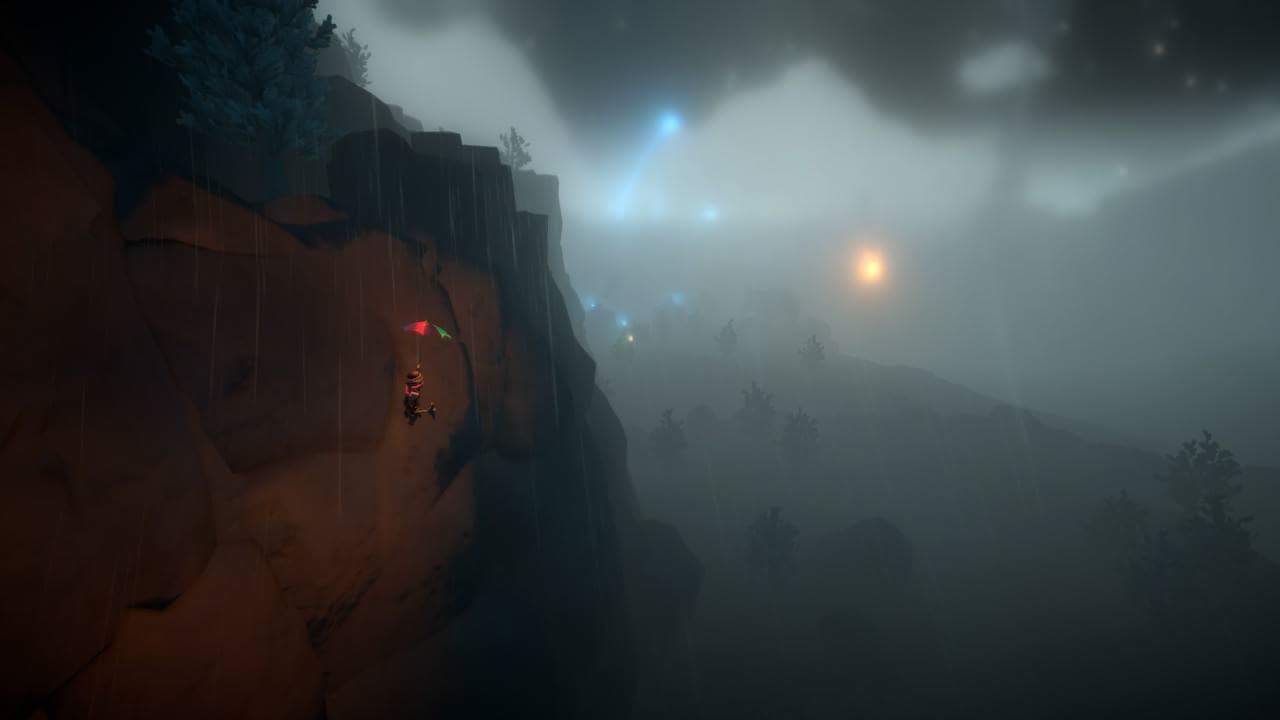A moody, rain-soaked scene from a video game captures the stillness of a dark, stormy night. The image reveals a gray sky shrouded with heavy black clouds, intensifying the downpour. On the left, a rugged cliff of light and dark brown rocks dominates the foreground. At the upper left corner, a dark-green tree adds to the scene's somber atmosphere. In the distance, a dense fog blankets the landscape, obscuring the silhouettes of distant trees. The fog merges seamlessly with the overcast sky, creating a hazy blend of grays. Piercing through the gloom, a warm, yellow light glows softly, providing a touch of warmth. Contrastingly, blue lights punctuate the scene—some twinkling in the sky, others illuminating the ground—adding an element of mystique to the desolate landscape.